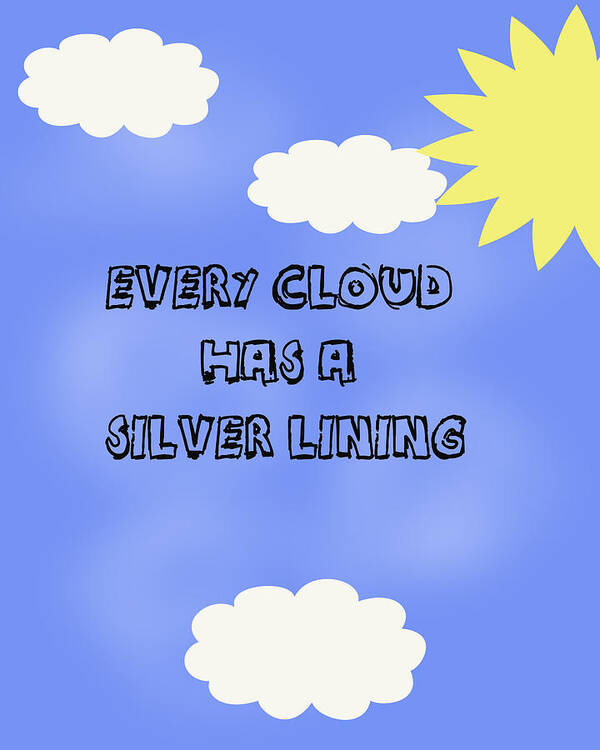This detailed description is of an inspirational poster with a childlike artistic rendition of a sky. The background is a gradient blue, featuring both lighter and darker blue hues that hint at distant clouds. Prominently on the upper right corner, there is a yellow sun with multiple triangular rays extending outward, although about half of it is cropped out of the frame. The sky is decorated with three puffy white clouds: two positioned at the top and one at the bottom center of the image. In the very center of the poster, large black print reads, "Every cloud has a silver lining." The background's blue also subtly fills the inside of the letters, adding a cohesive touch to the overall design. The simplicity and childlike drawing style of the elements make this poster a suitable piece for classrooms or libraries, aimed at delivering inspiration through its simple yet effective imagery and message.